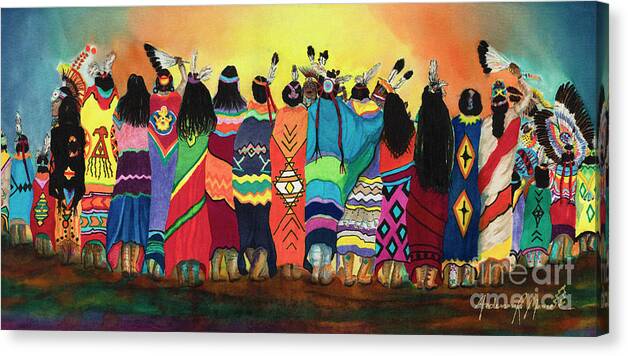This image is a photograph of a rectangular painting on canvas, set against a plain white background with a subtle light gray shadow along the bottom and right sides. The painting, approximately four inches wide and two to three inches high, vividly captures a group of Native American Indians standing around a bright fire against a dark blue sky. From left to right, the scene features around 20 individuals, both children and adults, all depicted from behind. They are dressed in traditional tribal clothing, with some wearing feathers in their hair or bound headbands, and one person on the far right sporting a full headdress. Each person is wrapped in colorful, patterned blankets: a striking yellow blanket with an orange, blue, and red threaded triangle design; a green, yellow, red, and black striped blanket; and a purple, black, and blue diamond patterned blanket among them. The ground beneath them blends vibrant oil colors of purple, green, orange, and brown. At the painting's center, they all gaze towards a radiant half-circle of yellow, encircled by orange rings, suggesting the glow of a fire or possibly a rising sun, with the colors transitioning to greens and blues on the periphery, emphasizing the rich cultural tapestry and the mesmerizing warmth of the scene.